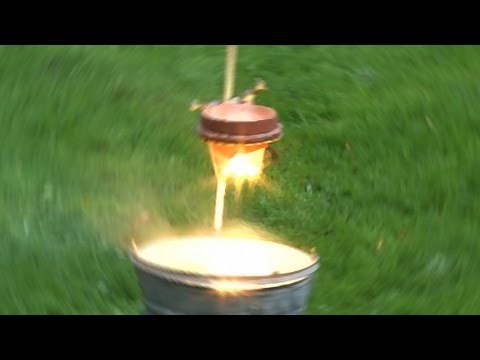The image depicts a metal pail, or tin can, standing in the grass, its simple handle reminiscent of those used for milk buckets. A pole, descending from the top of the image into the pail, supports a red-topped lamp that casts a striking orange light below. This illumination creates an effect akin to fire, causing an unusual and somewhat mesmerizing visual. The photograph is characterized by a distinct blurriness arranged in a circular pattern, making the center of the image clearer, while the borders – black stripes on both the top and bottom – accentuate this intriguing outdoor scene.